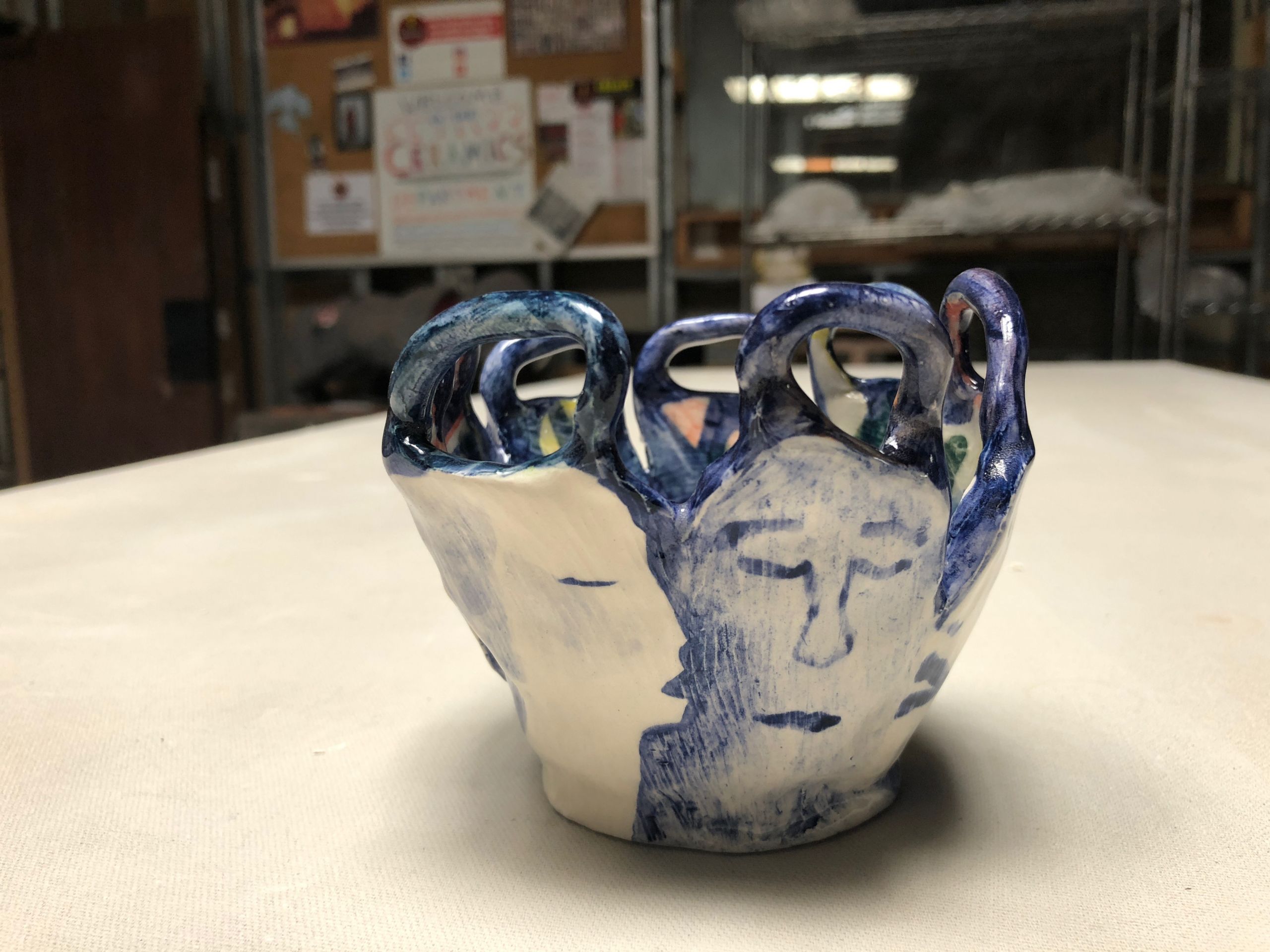The image features an intricately crafted ceramic piece displayed atop a large white table. The bowl-shaped object, primarily painted in shades of blue and white, boasts an array of at least six U-shaped handles adorning its top edge. Two distinct faces are meticulously depicted on its exterior. On one side, a rather crudely drawn blue face captures attention with bold strokes, exuding a sense of raw emotion or expression. On the opposite side, a more subtle white face with minimal blue accents represents a nose, mouth, and eye, seemingly gazing towards the blue face, creating an interactive dynamic between the faces. The piece sits in what appears to be a classroom or studio setting, evidenced by a blurred poster in the background that references ceramics, hinting at the handcrafted nature of the object. The overall ambiance suggests it may have been created or studied in a ceramics class environment.